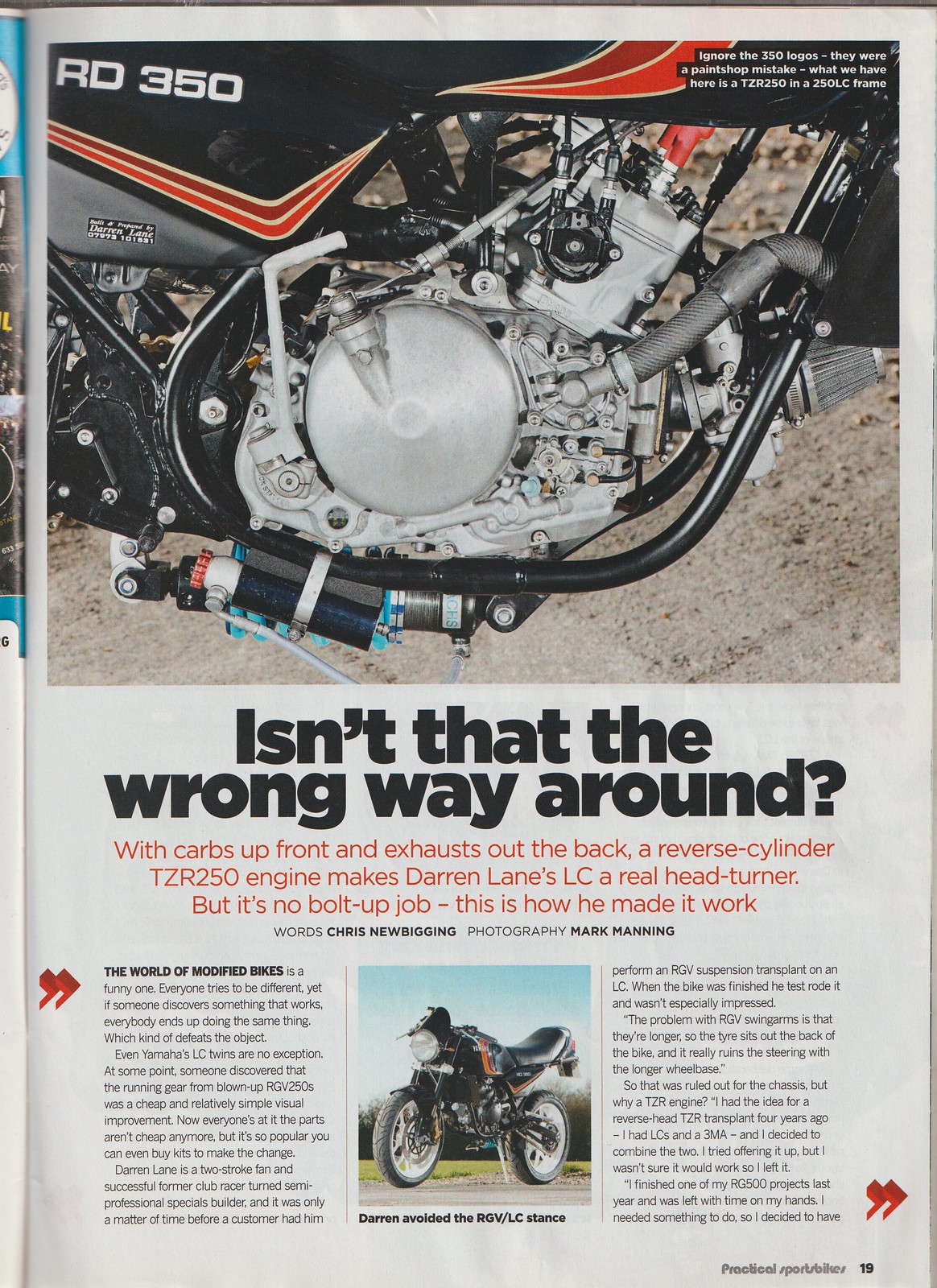This image is a scanned page from a magazine, specifically "Practical Sports Bikes," indicated by the text at the bottom right corner with the number "19" next to it. The top half of the page prominently features a close-up of a motorcycle engine, specifically a black and red TZR250 engine in a 250 LC frame. The headline, "Isn't that the wrong way around?" draws attention to the engine's unique configuration, with carbs positioned up front and the exhaust exiting out the back. This reverse cylinder setup makes Darren Lane's LC a real head-turner, although it’s explained that this is no simple bolt-up job—detailing the complexity of the modification. Underneath the image, the article provides further description and elaborates on how Darren avoided the RGV LC stance, mixing practical advice with his innovative approach. The text, credited to writer Chris New Bigging and photographer Mark Manning, is divided into two columns flanking another image of the bike, offering an informative glimpse into the meticulous work and creativity involved in this motorbike modification.